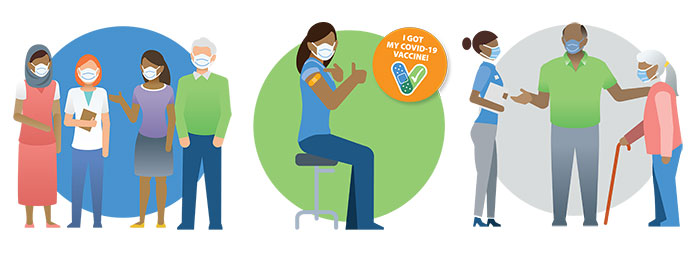This infographic, presented in three side-by-side segments with a white background, encourages COVID-19 vaccination. The left segment features a blue circle backdrop with four faceless, corporate-styled figures, all wearing masks. From left to right, there's a Muslim woman in a pink dress with a headscarf, a red-haired woman in a short-sleeve white blouse and blue pants holding a notebook, a Black woman in a purple and gray dress with long dark hair appearing to talk, and an older man with gray hair in a green long-sleeve shirt and blue pants. The central segment, set against a green circular background, showcases a woman of dark complexion seated on a stool, dressed in blue pants and a white-blue shirt with rolled-up sleeves, revealing a band-aid on her arm. A smaller orange circle beside her indicates she received the COVID-19 vaccine. In the right segment, with a gray circle backdrop, an older balding Black man stands, seemingly in conversation with a nurse. He places his hand on the shoulder of an older woman with gray hair in a ponytail, who uses a cane. The nurse, wearing a blue top and gray pants, completes the scene, emphasizing healthcare support and vaccination.